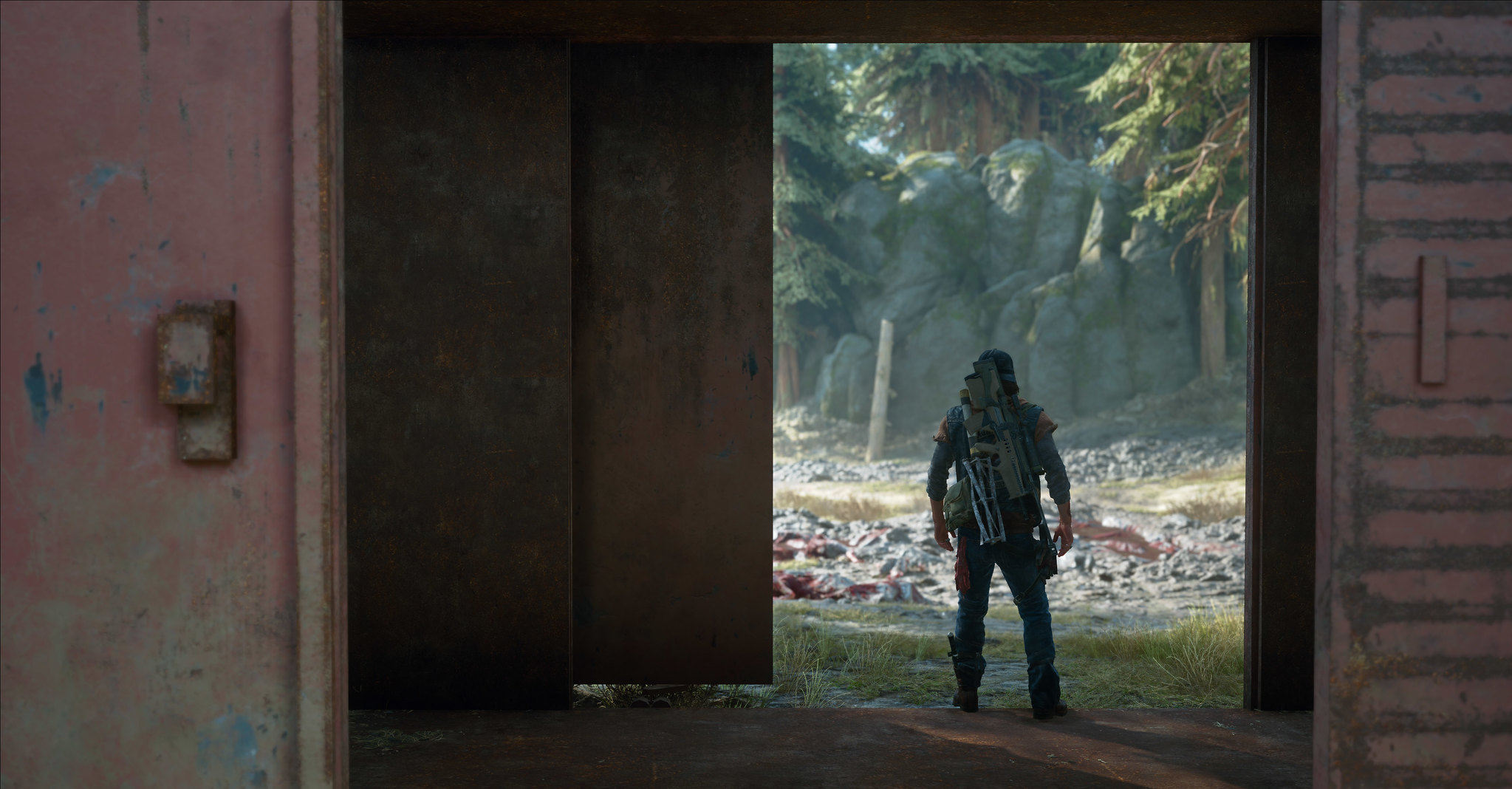In this video game cutscene, the protagonist, whose gender is indeterminate from the angle, stands with their back to us inside a structure that closely resembles a train carriage, identifiable by its two side doors with one partially open. The building, painted in a rich reddish-brown or maroon hue, frames the character who is armed with several types of firearms, including assault rifles, strapped to their back. They are dressed in blue jeans, sturdy boots, and a blue sweater, conveying a rugged and ready-for-action appearance. The character gazes intently out into a picturesque wilderness scene featuring tall pine trees, patches of snow, and verdant grass. Dominating the horizon is a large rock formation, possibly part of a mountain, adding a dramatic and natural backdrop to the scene. The interior of the structure remains largely unseen, with the sole focus being the armed character and the vast, nature-rich vista they are engrossed in.